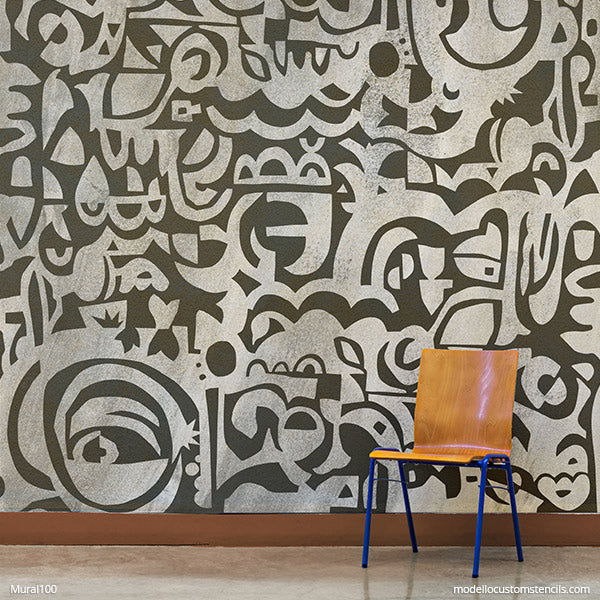In the image, there is a detailed view of an interior room, showcasing a floor covered in beige tiles complemented by a brown baseboard along the bottom of a wall. The wall itself is adorned with a geometric, black and white pattern that could be an intricate wallpaper or possibly a large, freestyle stencil design. This pattern is filled with various nondescript shapes and symbols, including curves and perhaps some crescent moons, creating a visually complex and artistic backdrop.

A wooden chair with a brown back and seat, all made from a single piece of wood, sits prominently in the lower right portion of the image. This chair is supported by a blue metal frame that includes the legs. 

At the bottom of the image, there is text. On the left side, it reads "Mural 100," while on the right, it says "ModeloCustomerIndex.com," though one voice suggested it could also be "ModeloCustomStencils.com." The combination of the intricate wall design and the distinctive chair creates a visually stimulating and artistic scene within the room.